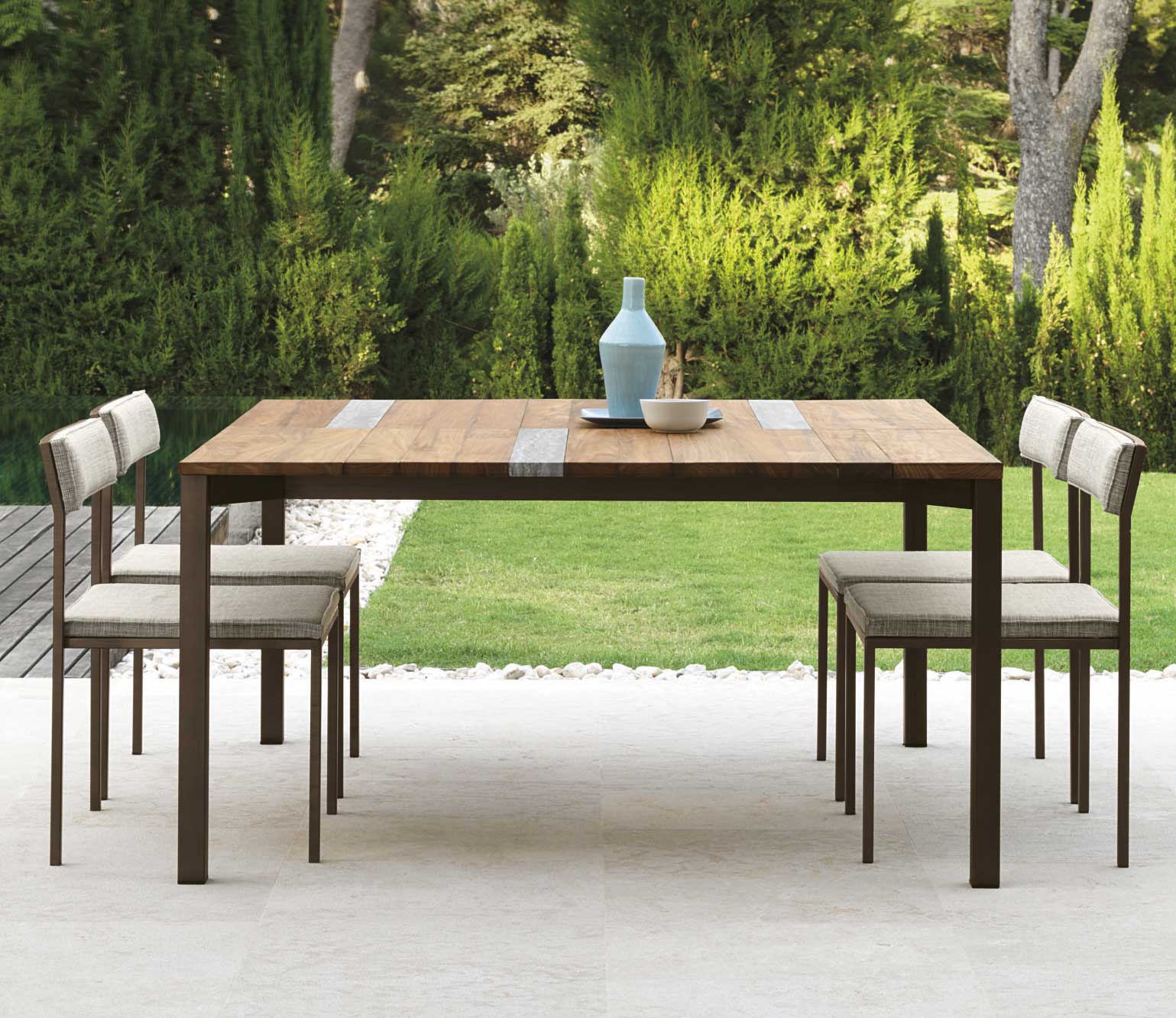This is an outdoor, color photo capturing a square wooden table with a unique pattern of orange and grey toned boards, resembling bricks, interspersed with occasional grey boards. The table, situated on a white-paved patio edged with white rocks, is accompanied by four matching brown chairs—each featuring thin legs and padded seats and backs in tan. On the table sits a light blue vase at the center and a white bowl placed adjacent to it. This setup is surrounded by a meticulously maintained lawn of short-cut grass. Beyond the lawn, there is a layer of assorted trees, including some conifers, adding a natural and lush backdrop to the setting.